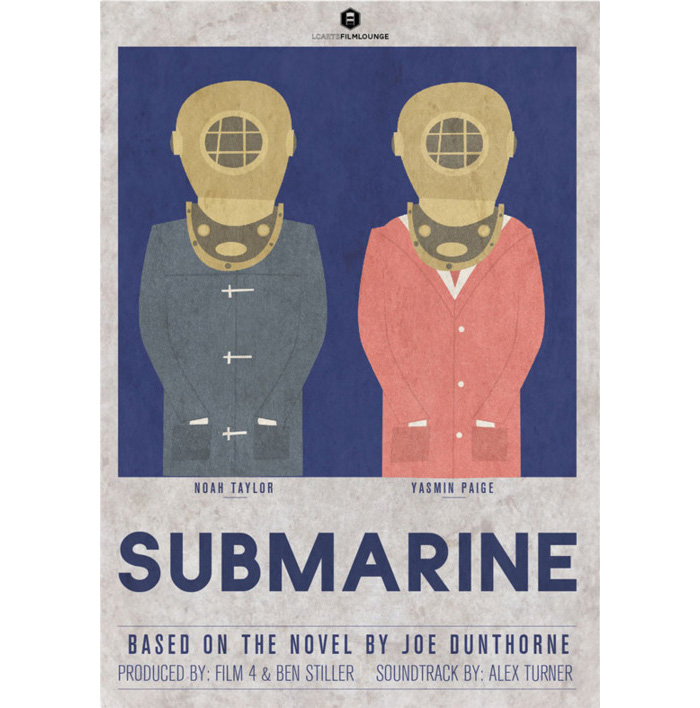The movie poster for "Submarine," based on the novel by Joe Dunthorne, features two people at its center, each wearing an old-fashioned metal diving helmet that obscures their faces. The diving helmets are brown with screened face guards and extend past their necks. The person on the left dons a full-length gray coat, while the person on the right is dressed in a full-length pink coat. At the top of the poster, somewhat obscured, it appears to read "L Cart 2 Film Lounge," possibly with an accompanying logo. Below the person in the gray coat, the name "Noah Taylor" is displayed, and beneath the person in the pink coat, the name "Yasmin Paige" is written. Underneath their names, the title "Submarine" is prominently presented in big blue letters against a light blue background. Below the title, it reads "Based on the Novel by Joe Dunthorne," followed by "Produced by Film 4 and Ben Stiller" and "Soundtrack by Alex Turner."